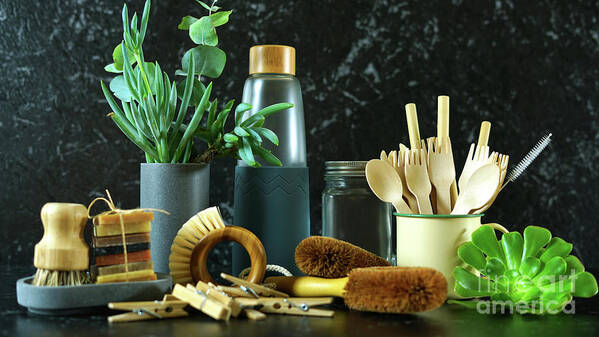The image displays a collection of kitchen and cleaning items arranged on a dark-colored countertop, set against a dark bluish-green wall. Dominating the scene is a large bowl filled with a variety of utensils, including wooden, or wood-like, spoons and forks. To the left, there are two brushes with wooden handles; one has round white bristles, suitable for scrubbing plates, while the other is a longer, narrow brush designed to clean inside cups. Nearby, a cluster of plastic spoons and sporks is housed in a white cup. Scattered across the counter are several clothespins and thin bars of soap or wax, neatly tied with string. A dark blue vase or cup holds a green plant, resembling a small cactus, adding a touch of greenery to the setting. Additionally, there is a mason jar with a wooden lid, potentially containing water, contributing to the assortment of items. The scene is completed by the sight of a black wall in the background, speckled with white, giving it a marble-like appearance, and the words "In-Cart America" subtly visible in the bottom right corner.